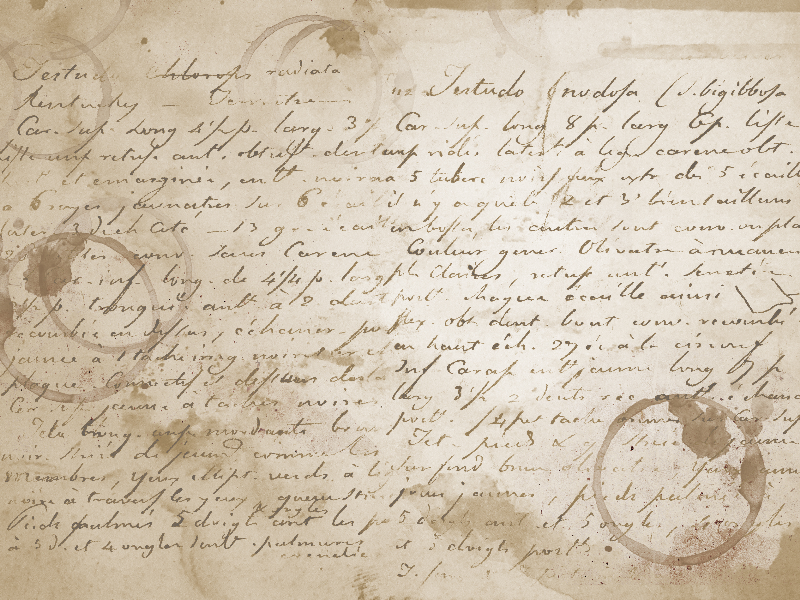The image portrays a very old and weathered piece of parchment or vintage paper, filled with cursive writing. The paper is a tarnished golden brown, heavily stained with multiple overlapping circular rings and dark blotches — indicative of old coffee or tea cups. The rings vary in size and intensity, concentrated mostly on the left side and the center, with prominent stains including a large coffee stain in the lower right and several overlapping rings towards the middle and left sides. The text, written in faded black or dark brown ink, is difficult to read due to the aged condition and potential language barrier. The writing spans nearly the entire surface, consisting of around 12 lines, and the most distinguishable word is "testudo," found just to the right of the middle at the top. Overall, the document gives the impression of having been written centuries ago, possibly with a quill, and now appears almost illegible due to wear, fading, and extensive staining.